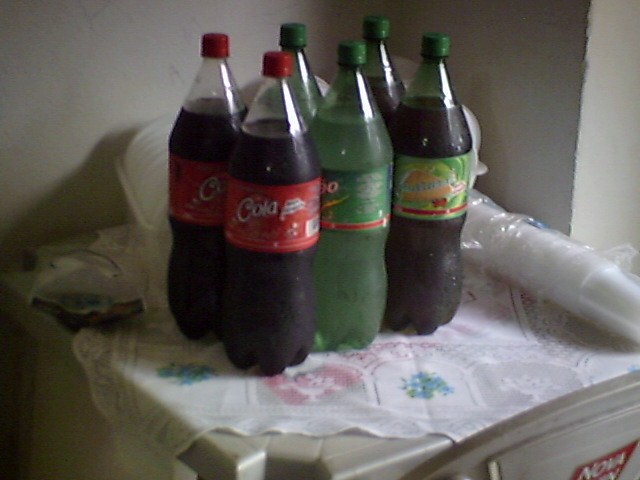In a dimly lit room, a photograph captures a small table against a plain white wall. The table is covered with a white tablecloth adorned with floral prints. On the tablecloth, to the left, there's a stack of white plastic cups wrapped in clear plastic. Center-stage on the table are six unopened soda bottles arranged in two rows. Two bottles with red caps and red labels display the familiar white 'Cola' text, containing a dark brown liquid. Next to them, two bottles of Sprite have light green liquid and green caps with matching light green labels. In the back, partially obscured, are two more bottles with green caps. These have a darker liquid, potentially a fruit-flavored soda as suggested by the images of berries and orange slices on their green, red, and orange labels. The edge of the image hints at a red label on a piece of furniture or cooler marked ‘Nova’, though the rest of the text is not visible.